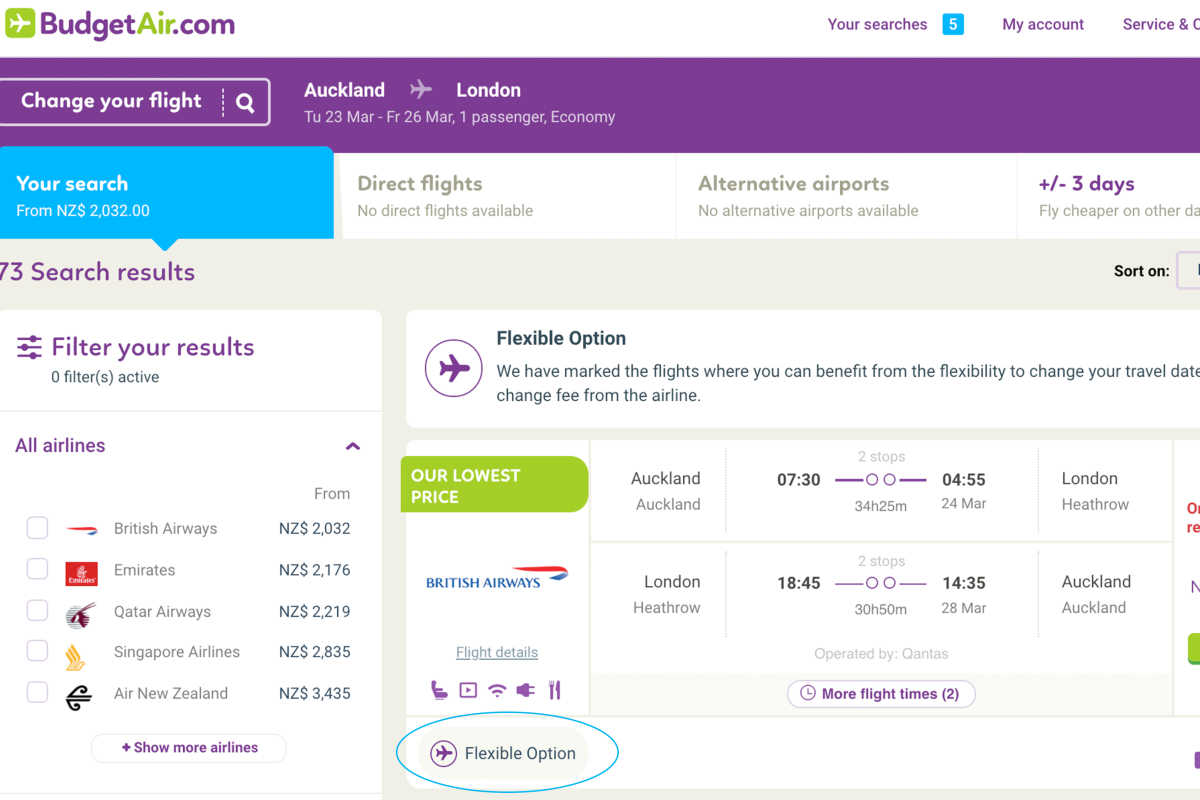The image depicts a webpage from budgetair.com, an airline booking website characterized by its white, green, and purple color scheme. At the top of the page is a "Change Your Flight" button. The visible flight details are for a trip from Auckland to London, scheduled from Tuesday, 23rd March to Friday, 26th March, for one passenger in economy class. 

The display indicates that no direct flights are available, nor are there alternative airports. There is an option to adjust the travel dates by plus or minus three days to potentially find cheaper flights. A section called "Your Search" shows the current search details originating from New Zealand, with the figures 2000 and 2032, and indicates 73 search results.

On the left side of the screen, there is an option to "Filter Your Results," which currently has zero active filters. A list of airlines is displayed, including British Airways, Emirates, Qatar Airways, Singapore Airlines, and Air New Zealand.

To the right, the departure and return trip timings are shown: the outbound flight from Auckland to London is from 07:30 to 04:55, and the return trip from London to Auckland is from 18:45 to 14:35. Additionally, there is a "Flexible" option that is highlighted or circled, suggesting that the user is interested in flexible travel dates.